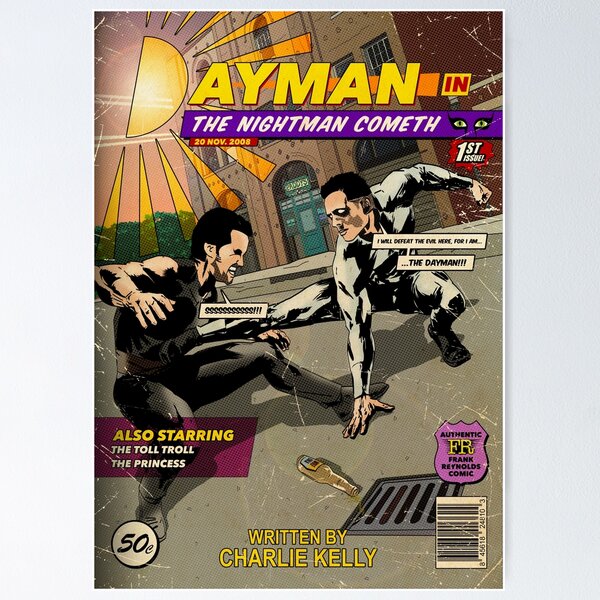The image is a detailed cover of an old-looking comic book titled "Dayman," from the episode "The Nightman Cometh" of the TV show "It's Always Sunny in Philadelphia." The vibrant cover features bright yellow text at the top that says "Dayman," with sun rays emanating from the first letter. Below the title, it reads "Dayman in The Nightman Cometh" written by Charlie Kelly. The setting is a neighborhood scene in front of Paddy's Pub, which is owned by the characters in the show. Two cartoonishly muscular men, appearing to be Charlie Kelly and Dennis Reynolds dressed up as superhero Dayman and his nemesis, Nightman, are in dramatic fighting poses. The Dayman character is wearing a tight, white bodysuit and declares, "I will defeat the evil, for I am the Dayman." The background includes detailed elements like a beer bottle next to a gutter, adding to the authenticity of the scenery. Below the main art, there's a fake publish date, "November 20th, 2008," and a price of 50 cents, emphasizing the whimsical and nostalgic nature of the cover.